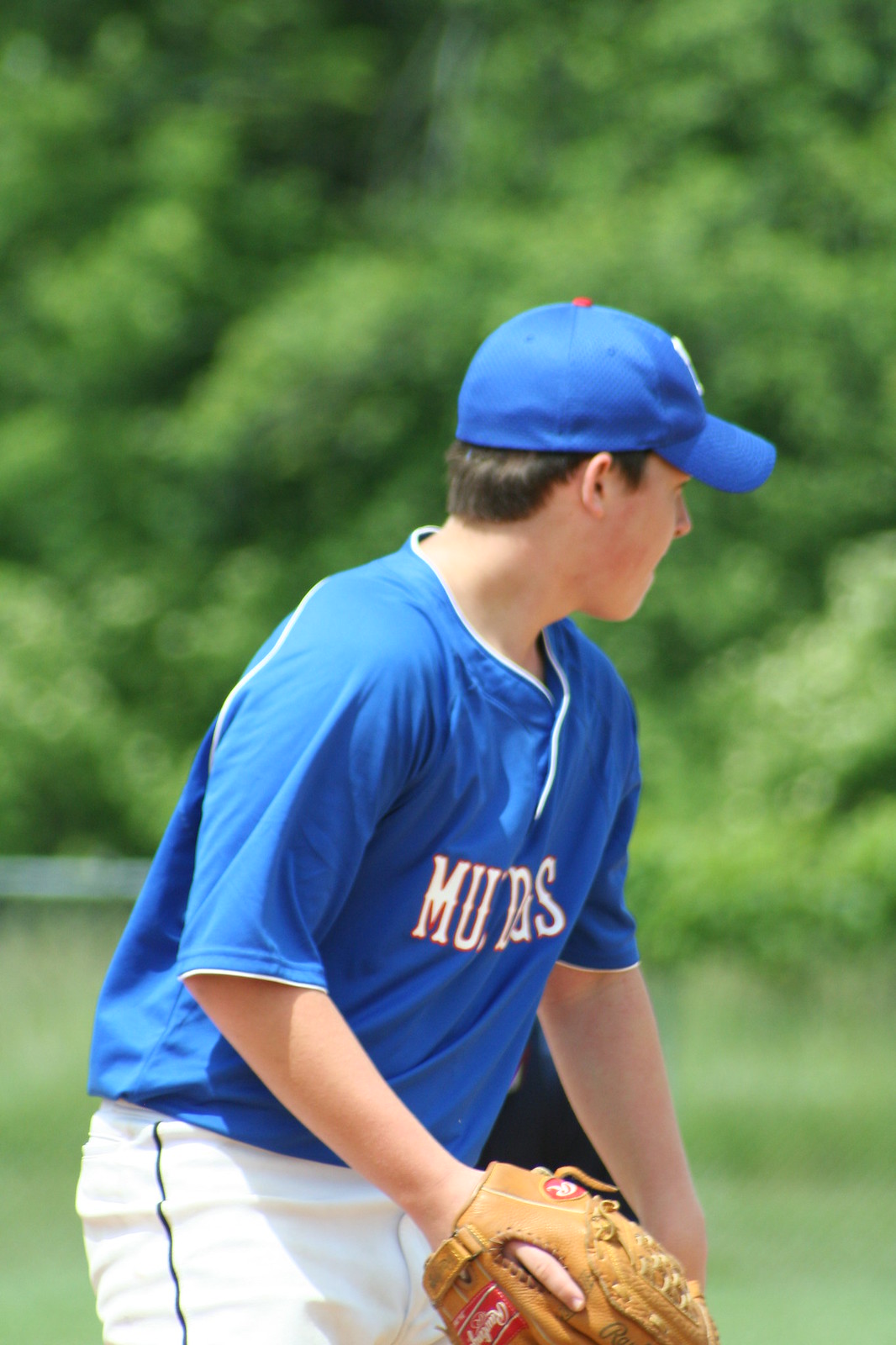This low-resolution color photograph captures a young adolescent boy standing outdoors in the bright sunshine, dressed in a blue baseball uniform. He is wearing a blue shirt with white text across it, which features white piping around the collar and the edge of the sleeves, and is reminiscent of a classic baseball shirt. Complementing his top, he has white pants with a thin dark green stripe running down the side from the hip. Completing his outfit is a blue baseball cap with a small red dot on top, which sits firmly on his head, partially covering his short brown hair. In his right hand, he holds a light brown leather baseball glove that has a red tag with white writing on it. The boy stands towards the right side of the image, his head turned away and looking towards the distance to the left. The backdrop is a blurred mix of trees and sunlight, providing an indistinct yet warm and summery feel to the scene. His stance and attire suggest he is involved in a baseball game, possibly in a pitching position, although no other players are visible in this shot.